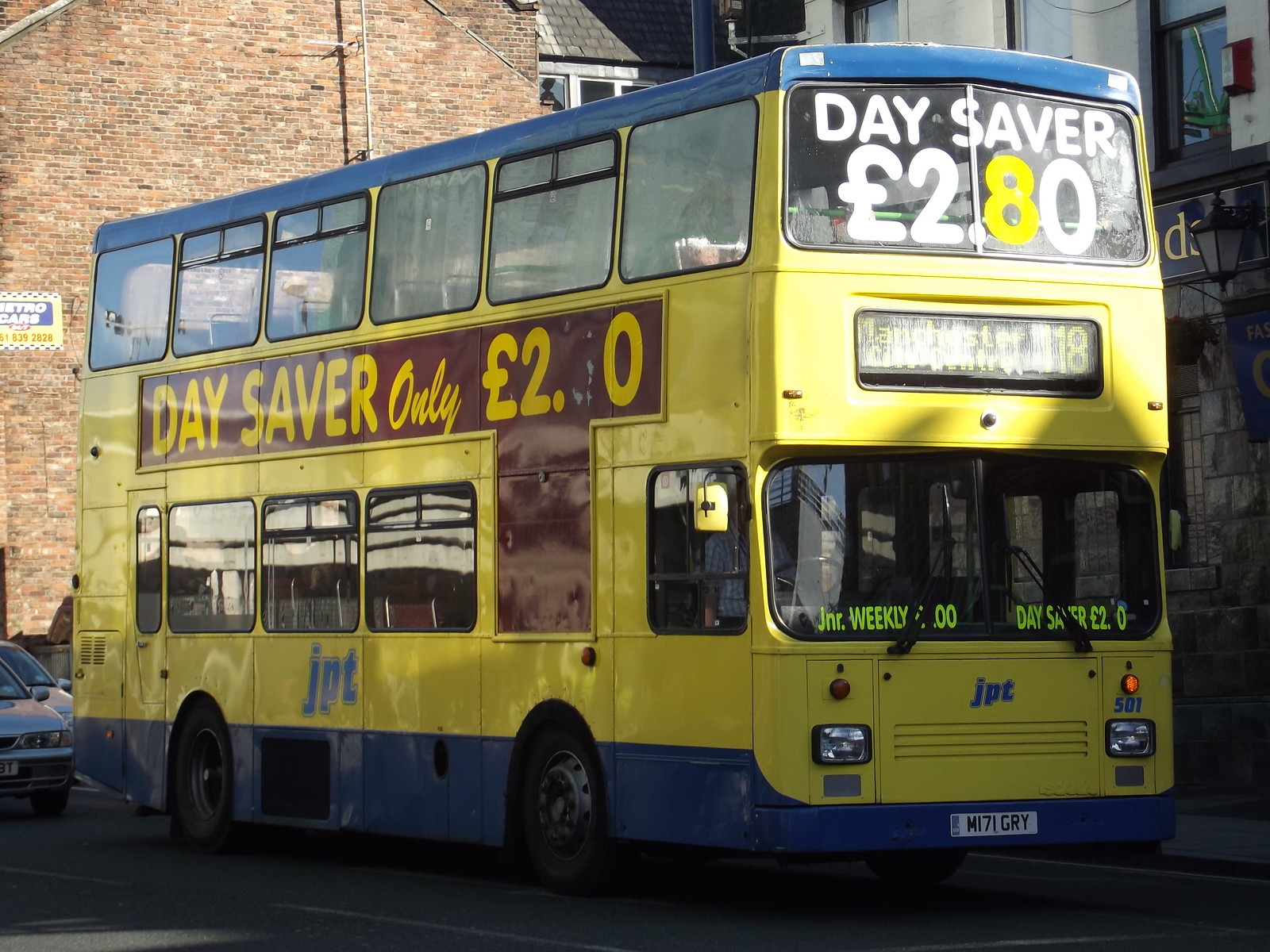This vibrant photograph captures a yellow double-decker bus with blue accents driving along a bustling road. The bus's distinctive design features six windows on the top deck and five on the lower deck, with two windshields for the driver and passengers. The left side of the bus displays text promoting a "Daysaver" fare for "only £2.00," although some digits appear to be physically altered, suggesting a temporary price change. The front upper deck window repeats this information with "Daysaver £2.80," where the digit "8" stands out in yellow. The bus proudly bears the JPT logo on both its side and front. In the background, smaller cars follow the bus, and a series of brick buildings line the street. Portions of the bus are bathed in light, creating a contrast with the shaded areas, adding depth and highlighting the dynamic city scene.